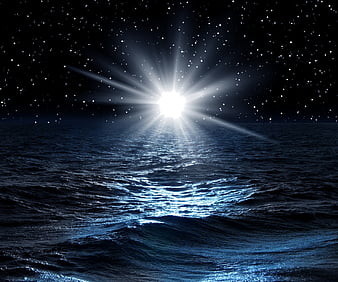This is a small, square image, appearing to be a stylized photograph or drawing of an ocean scene at night. The sky is dark, filled with numerous tiny pinpoints of light representing stars. At the center of the image, there is a bright, white glow with radiating beams of light, suggesting a moon, although its brightness resembles that of the sun. This luminous body is situated just over the horizon, casting a reflective, shimmering light on the surface of the deep blue ocean. The water is depicted with large swells and waves, creating a dynamic interplay of light and shadow across its surface. The bright, illuminated trough in the middle contrasts sharply with the much darker waves on either side, enhancing the overall dramatic effect of the scene.